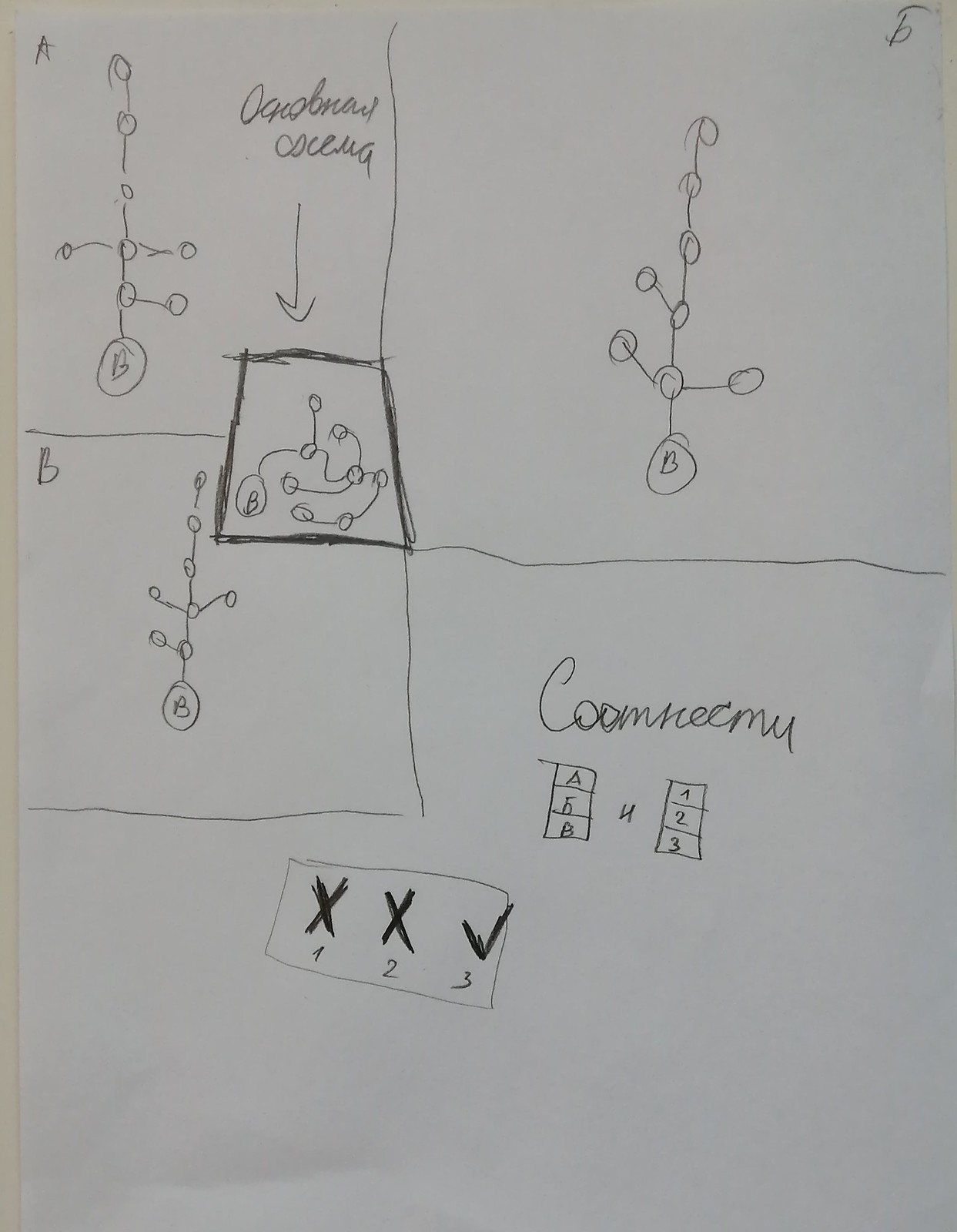This close-up image shows a detailed diagram drawn with black ink on white paper, showcasing what appears to be a complex chemical or biological structure. The diagram is segmented into parts labeled A, B, and C, each depicting a tree-like structure with interconnected circular lines. The main structure, labeled D-Q-O-L-N-A-W-C-O-C-E-U-G, features a central trunk with branches forming dashed, circular connections to various segments.

An arrow points downward from these labels to a prominently bordered box, illustrating a variation of the circular lines, which are curved and arced, converging to a circle with the letter "B" at its center. This larger circle is situated at the base of the central line, forming a molecular-like structure. The section labeled "B" mirrors "A" but with different branch connections.

To the right of the structure, additional labels read A-F-B-N-H-A-2-3. At the bottom center, enclosed within a box, it is marked "1-2-3." Notably, bold black ink marks an "X" over "1" and "2," while a checkmark is placed over "3," indicating a specific endpoint or conclusion.